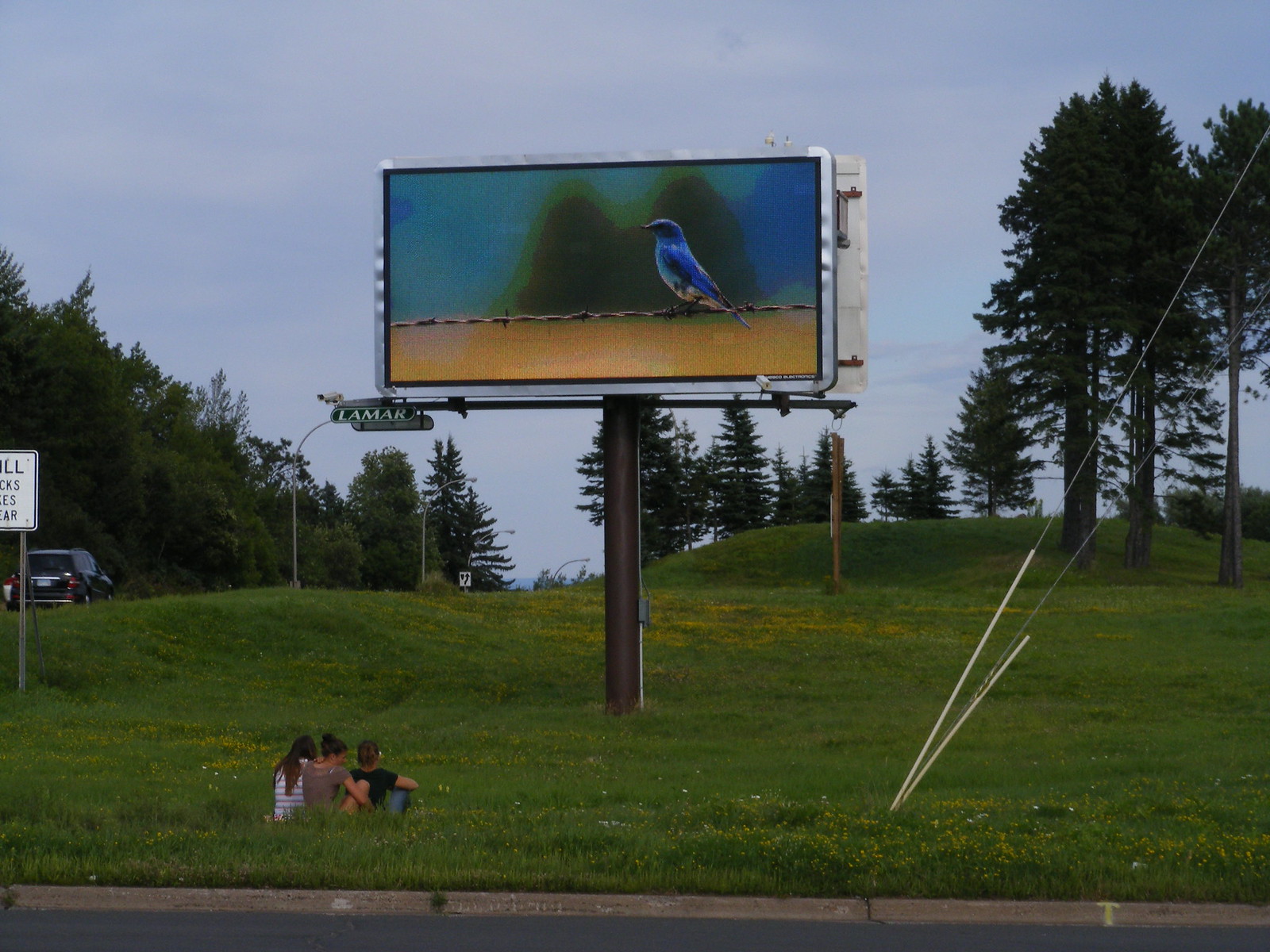In this photograph, three young women are seated in a lush, green grassy field with occasional yellow flowers, gazing up at a large digital billboard mounted on a dark brown metal pole. The billboard, surrounded by a silver border, displays a clear image of a small blue bird perched on a slender barbed wire fence. Below the bird, the background becomes indistinct with blurred brownish hues, possibly indicating crops.

The women are huddled together on the grass, with their knees pulled up to their chests. To the left, one woman with long hair wears a gray and black striped shirt. Next to her, a woman with short hair is dressed in a taupe-colored t-shirt, and on her right is another short-haired woman in a black shirt and blue jeans.

In the background, a tree line comprised of tall pine trees stretches across the field, tapering off into an open space before resuming. The sky above is a rich, darker blue interspersed with light gray clouds on a somewhat muggy day. Telephone wires, wrapped in white plastic at their base and transitioning to silver cables, can be seen extending up from the right side of the image.

To the left of the women, partially visible among the grassy expanse, a dark gray SUV drives down a nearby street. A green street sign with white text reads "Lamar." Just beyond the car, an expanse of trees and slight hills complete the backdrop, enhancing the serene, natural ambiance of the scene.